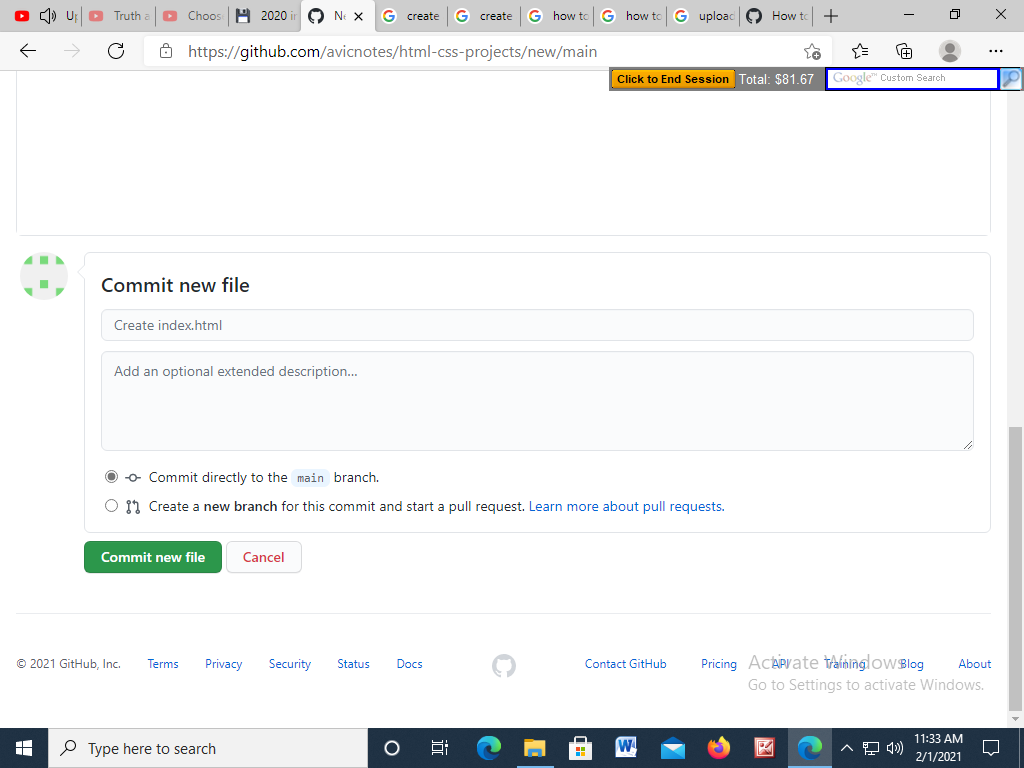A screenshot of a typical browser window on a Windows operating system.

The taskbar at the bottom features the Windows icon on the left, enabling access to files and applications like Google and Mozilla Firefox. There is also an icon for Microsoft Word, the system time, volume control, and the date. 

At the top of the screen, there are around ten open tabs within the browser, with the fifth tab from the left being the active one, indicated by its white background while others are grayed out. On the top right, the minimize, maximize, and close buttons are visible. 

Currently displayed on the browser is a GitHub page, as shown by the URL in the search bar. To the left of the search bar are navigation arrows and a refresh button. There is also an option to save the page to favorites. 

Below the search bar, a notification bar includes a yellow button labeled "Click to find session," the text "total: 81.67," and another Google custom search bar. 

Further down is a mostly empty white area, with another white box labeled "Commit new file." Near this box is an icon adorned with green squares. Below this section, there is a text field labeled "create index.html" and another field titled "add additional extended description."

Within this form, the default option "Commit directly to the main branch" is selected and grayed out, with an alternate option to "create a new branch for this commit and start a pull request." At the bottom, there’s a green "Commit new file" button and a "Cancel" button to its right.

The page footer includes links to GitHub's terms, privacy, security, status, docs, contact information, pricing, blog, about, and training sections, along with a mention of "GitHub 2021, Inc."